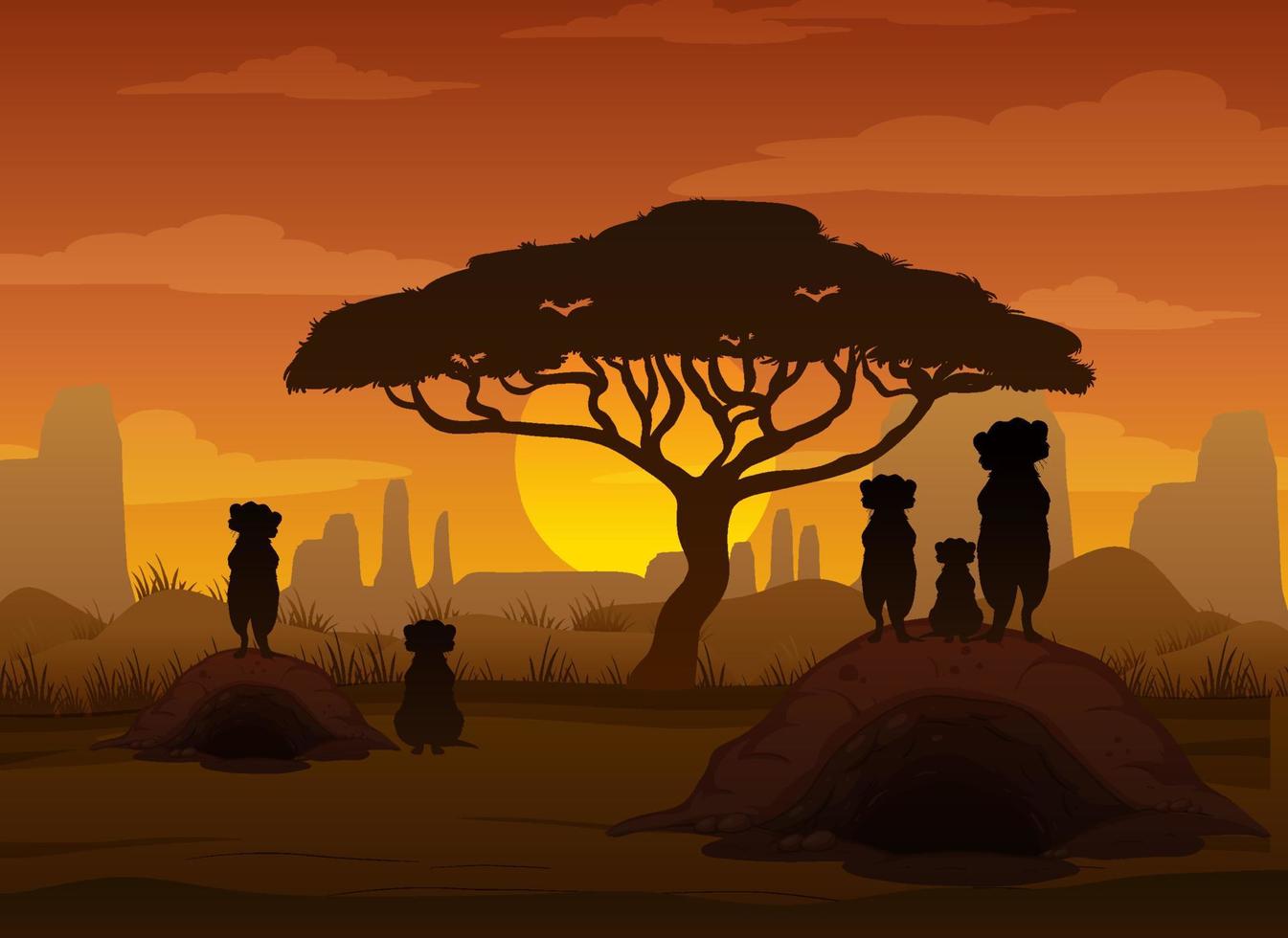The image is a cartoony painting of an African desert landscape. The ground is predominantly brown and green, featuring two prominent mounds of soil on either side. On the right mound, there are three animals, resembling meerkats, two of which are standing while a smaller one is between them. On the left mound, another meerkat stands alongside a seated one. These animals are seen in silhouette, facing forward, highlighting their outlines without detailed body features. In the middle ground, a distinctively wide-canopied African tree stands prominently, and behind this tree, light brown human buildings can be seen in the distance. The sky is a gradient of red and yellow, with the large yellow sun positioned near the horizon, casting a warm glow. Darker orange clouds pepper the sky, enhancing the sunset ambiance.